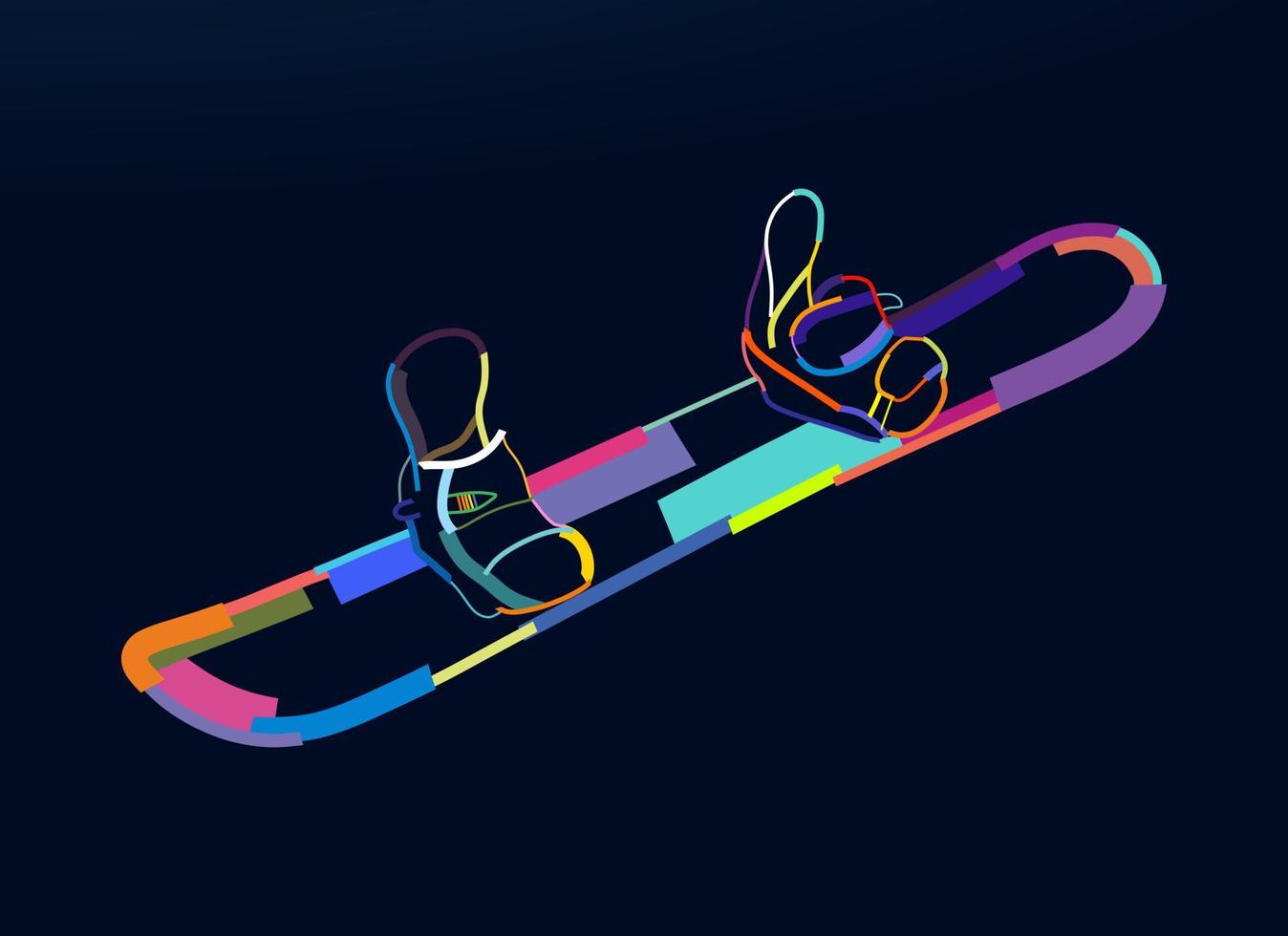This illustration showcases an abstract, contemporary depiction of a snowboard and its attached boots, both prominently outlined against a dark backdrop, either black or dark gray. The snowboard, rendered in striking multi-colored outlines, features a dynamic palette including shades of pink, purple, light blue, dark blue, yellow, cyan, orange, light yellow, and various purples. The attached boots, one near the front and one towards the back of the snowboard, are similarly detailed with vibrant outlines, incorporating hues of red, yellow, and other colors. The image gives the impression that the snowboard is suspended in air, accentuating its modern and artistic style.